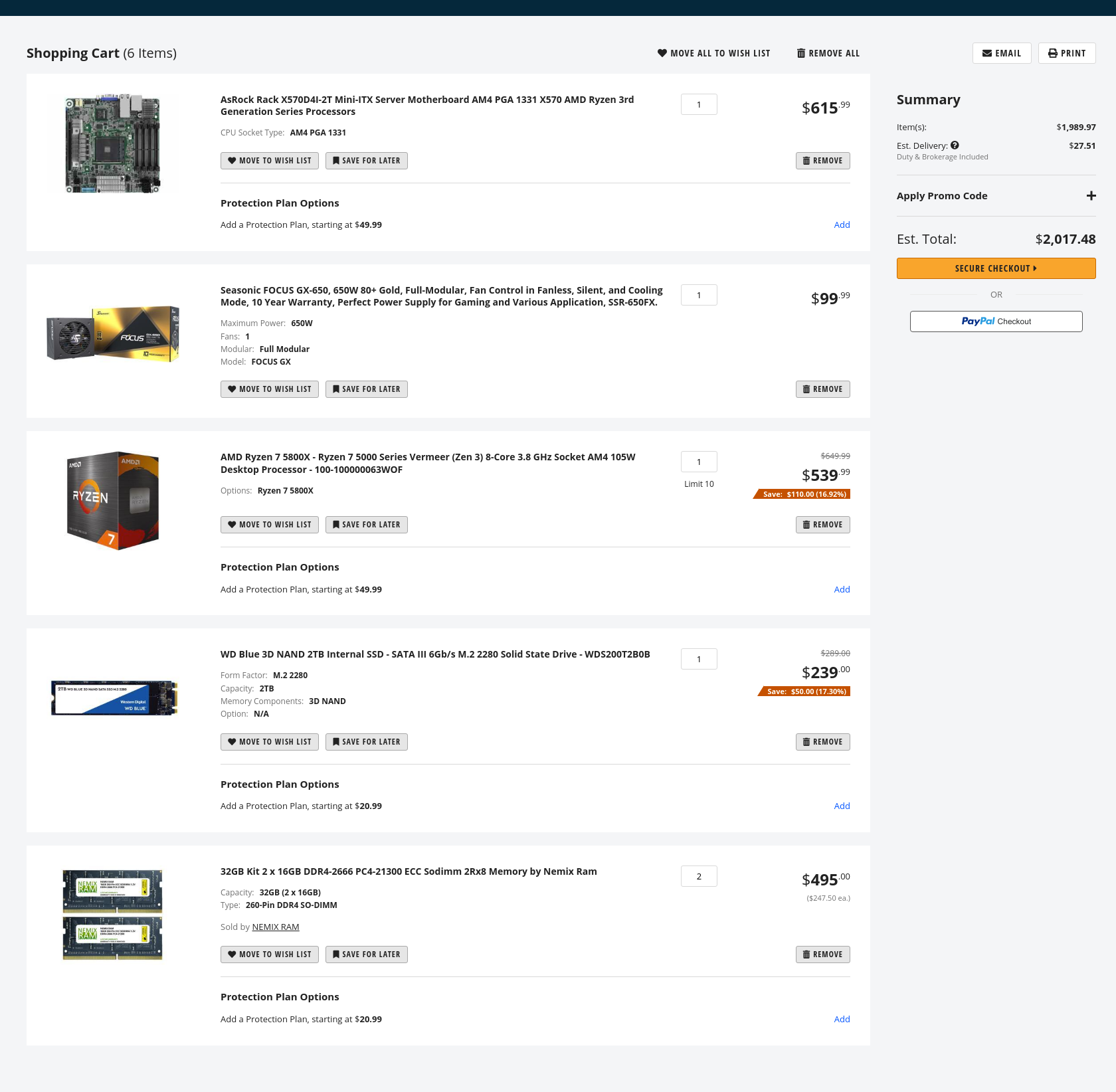In the image, a shopping cart on a web page displays computer components ready for purchase. The list contains five items, with small, difficult-to-read text on the right and images on the left. The top item is a motherboard priced at $615, identifiable by its detailed circuitry and slots. Following that, a component priced at $99 is visible, but its specifics are unclear. Further down, an AMD Ryzen series processor is listed at $539, clearly indicating its brand and model. Next, an SATA WD Blue 3D component, possibly a storage device, is priced at $239. The final item is a combination of components from a company called Mercenary, costing $495. Each item is visually represented to the left, but their descriptions require close attention due to the small text.